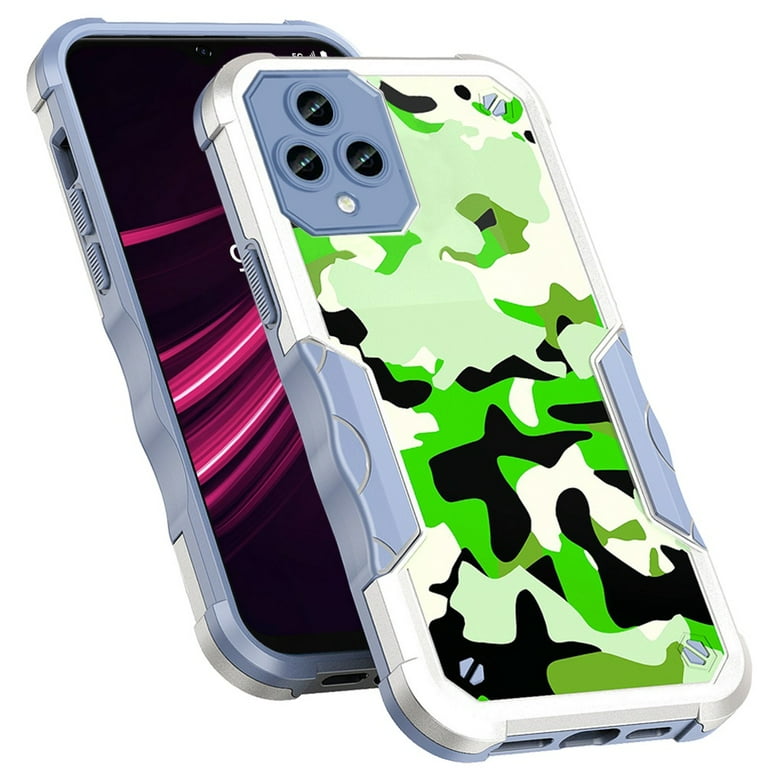The image depicts two cell phones stacked on top of each other, highlighting their intricate designs and protective cases. The bottom phone features a light blue edge, and its screen displays a black background adorned with red and white curved line patterns. The top phone also has a light blue edge with a touch of silver. It is positioned to be movable relative to the bottom phone. The bottom phone case is striking, showcasing a green, black, and white camouflage pattern with three camera lenses integrated into the top left corner, surrounded by three black holes. The case appears robust and protective, with thick frames that likely cushion the phones during drops. Near the bottom of the configuration, two speakers are visible, completing the detailed view of these well-designed devices.